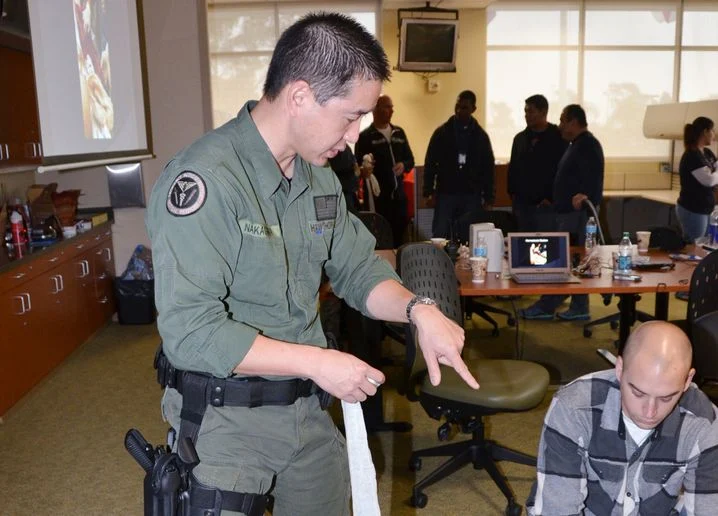This color photograph, taken indoors in a classroom or training center, features a man of Asian descent in the foreground wearing a green uniform suggestive of law enforcement or military affiliation. The man, who possesses short black hair, is equipped with a black utility belt and has an automatic handgun holstered on his right thigh. His uniform is adorned with various patches, including a medical patch and a United States flag, hinting at his EMS certification. He is holding a bandage in his right hand while pointing downward with his left hand, which has a watch on its wrist.

In front of him, a bald man wearing a gray, multi-patterned shirt is either kneeling or seated, possibly engaged in a medical certification test or training exercise, given his focused demeanor. Between them is a brown chair with a black back and a long brown table. 

The immediate background reveals a brown counter cluttered with various items, and drawers below the counter. Above the counter is a projection screen, partially visible on the left side of the image. Further back, a group of four or five people stands near a wall adorned with windows and a central television or monitor. The room is carpeted in a brownish-tan color, and additional details include a desk holding a laptop and some water bottles positioned further back on the right side of the image. This scene likely depicts a training or certification session for EMTs or paramedics, with the man in the green uniform serving as an instructor.